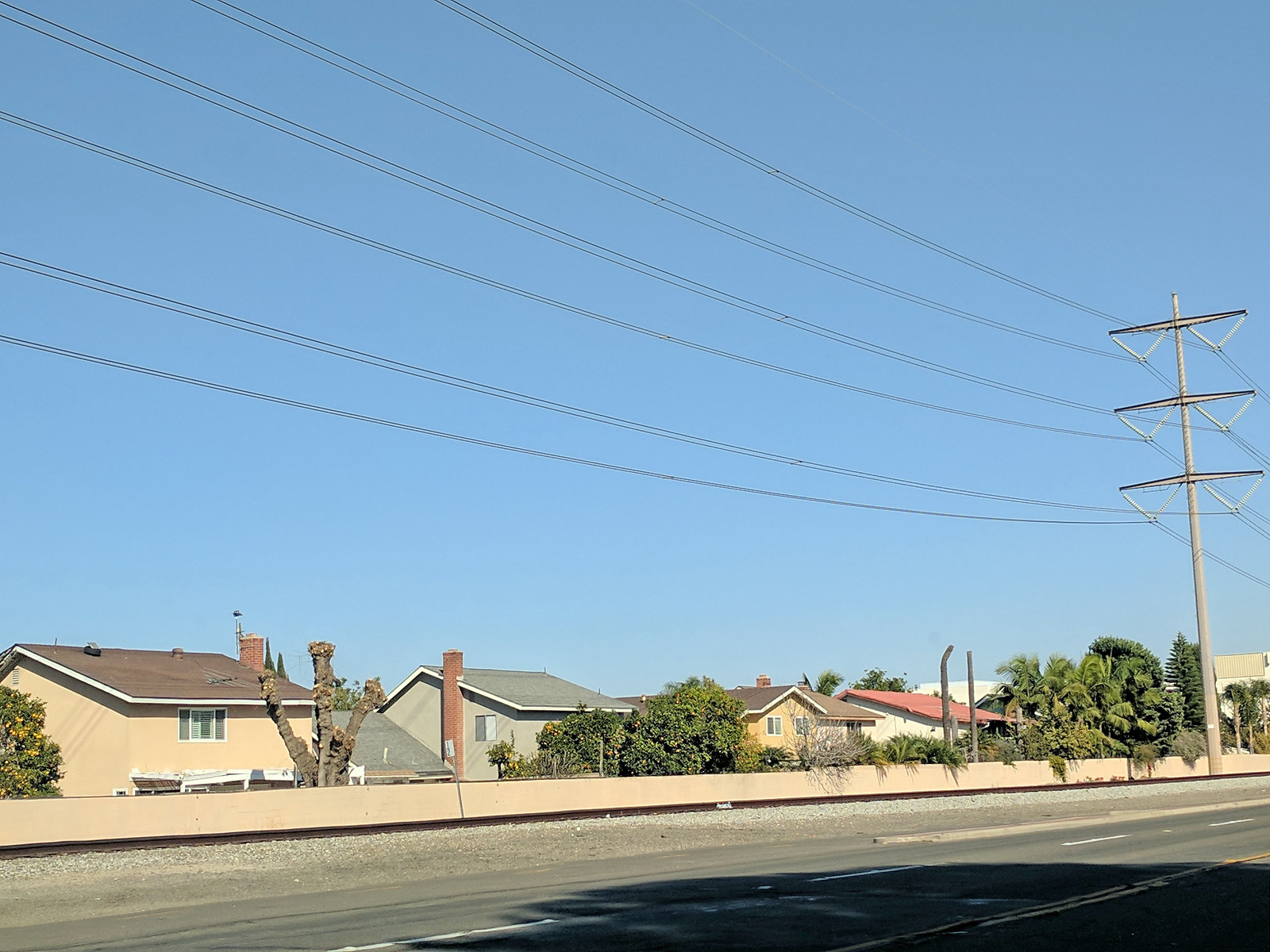This photo captures a busy suburban street that could be a small highway. The street itself is devoid of cars, but is bordered by a continuous concrete barrier. A utility pole stands prominently along the road, with utility wires stretching across the top frame of the image. The street is marked with the usual white painted road markings.

Beyond the barrier, a row of charming colonial-style homes lines the neighborhood. These two-story houses are painted in various colors: the first is a cream color with a brown roof, the second is gray with a matching gray roof, the third is a goldish yellow with a tan roof, and the fourth is white with a distinctive red roof. Each home is unique, adding a touch of character to the scene.

The backyards of these homes feature a mix of vegetation. Most trees are deciduous, though there is one palm tree and one coniferous tree in the mix. Notably, there is also a tree that appears to have been heavily pruned, now showing signs of new growth from its remaining trunks.

The sky above is a clear, light blue, indicative of a sunny day without clouds. The presence of a shadow in the foreground suggests that the time might be late afternoon.